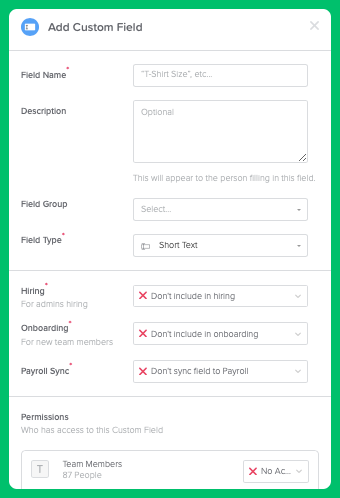The image displays a user interface for adding a custom field to a form. The interface is enclosed within a bright green border that is approximately half an inch thick. This green border frames a white to light gray background that contains various text fields and informational elements.

In the upper left corner, there is a blue circle with a white rectangle icon inside it, symbolizing the option to "Add Custom Field." To the right of this icon, the text "Add Custom Field" appears in gray, with a gray 'X' icon situated on the far right.

Below this, there is a label "Field Name" followed by an asterisk indicating it is a required field, accompanied by a text box labeled "t-shirt size." This is followed by a "Description" field marked as optional, which informs the user that whatever they input will be visible to the person filling out the form.

Further down, there is a "Field Group" selection box along with a "Field Type" dropdown menu, again marked with an asterisk to denote that it is required. The dropdown is currently set to "Short Text."

The interface also includes various options for integrations and permissions:
- "Hiring": There's a red 'X' indicating that this field should not be included in the hiring process.
- "Onboarding": Similarly, there's a red 'X' indicating exclusion from the onboarding process.
- "Payroll Sync": Another red 'X' specifies that the field should not sync with payroll systems.

At the bottom, under "Permissions," the form specifies who has access to this custom field. It notes that "Team members" comprising 87 people have access, followed by a red 'X' labeled "No AC."